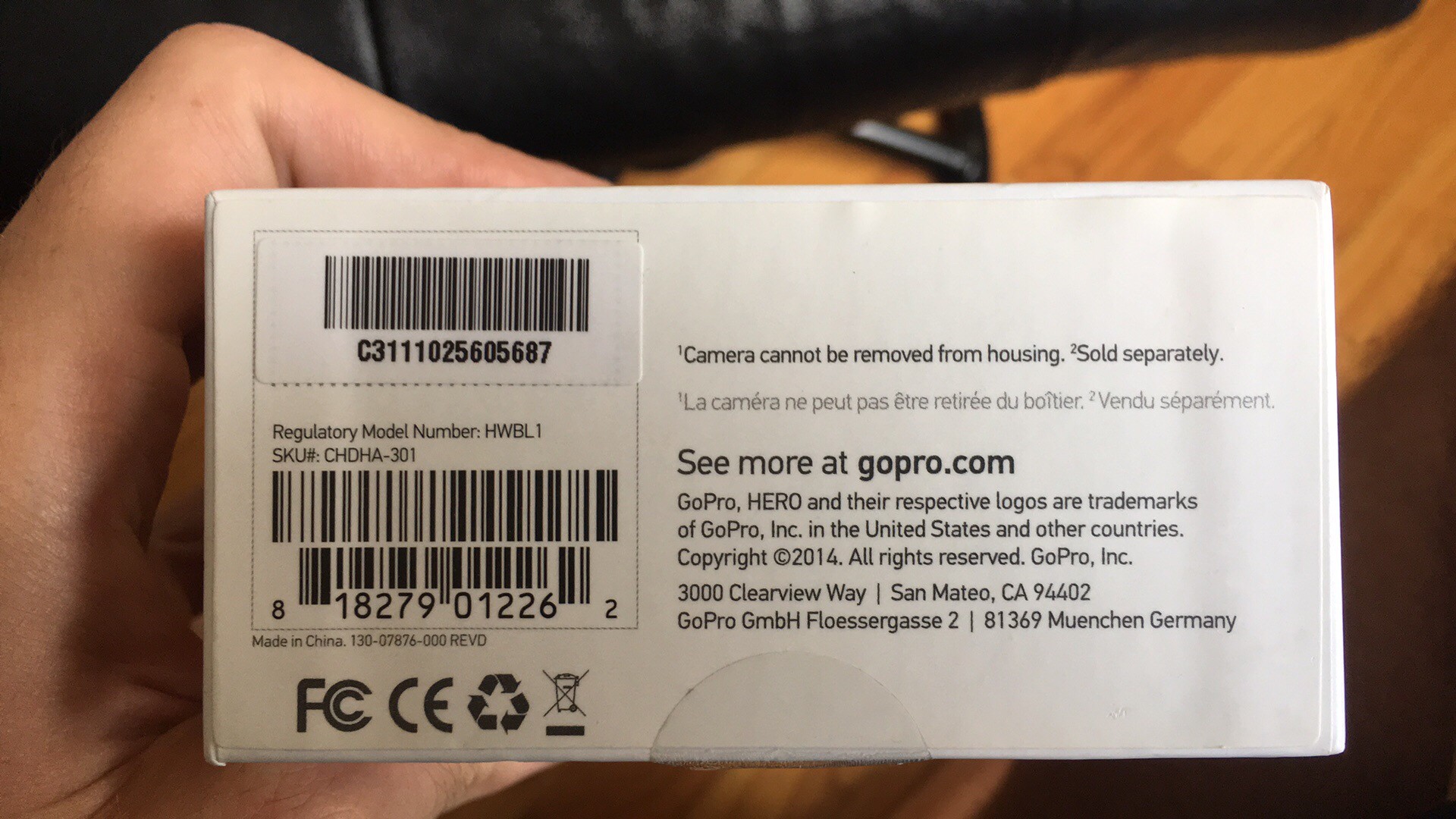The image features a high-quality photo of the bottom of a white GoPro box, held up by a person's hand. The bottom side of the box, prominently displayed toward the camera, includes various informational details. A QR code is positioned in a square in the center, accompanied by black text and symbols below it, such as the FC logo (with a smaller "C" inside the larger "C"), CE marking, recycling logo, and a trash can with an X through it. Additionally, the text indicates that the camera cannot be removed from its housing and is sold separately. The background of the image reveals a brown table with a black object, possibly a bag, stretching across the top, along with a wooden floor and part of a chair. The hand holding the box is visible on the left side, with the thumb partially wrapped around the box and the pointer finger bent at the knuckle, touching the top left corner of the box. The text also includes GoPro's website, contact information, address, and a barcode, denoting the GoPro Hero and its respective trademarks.